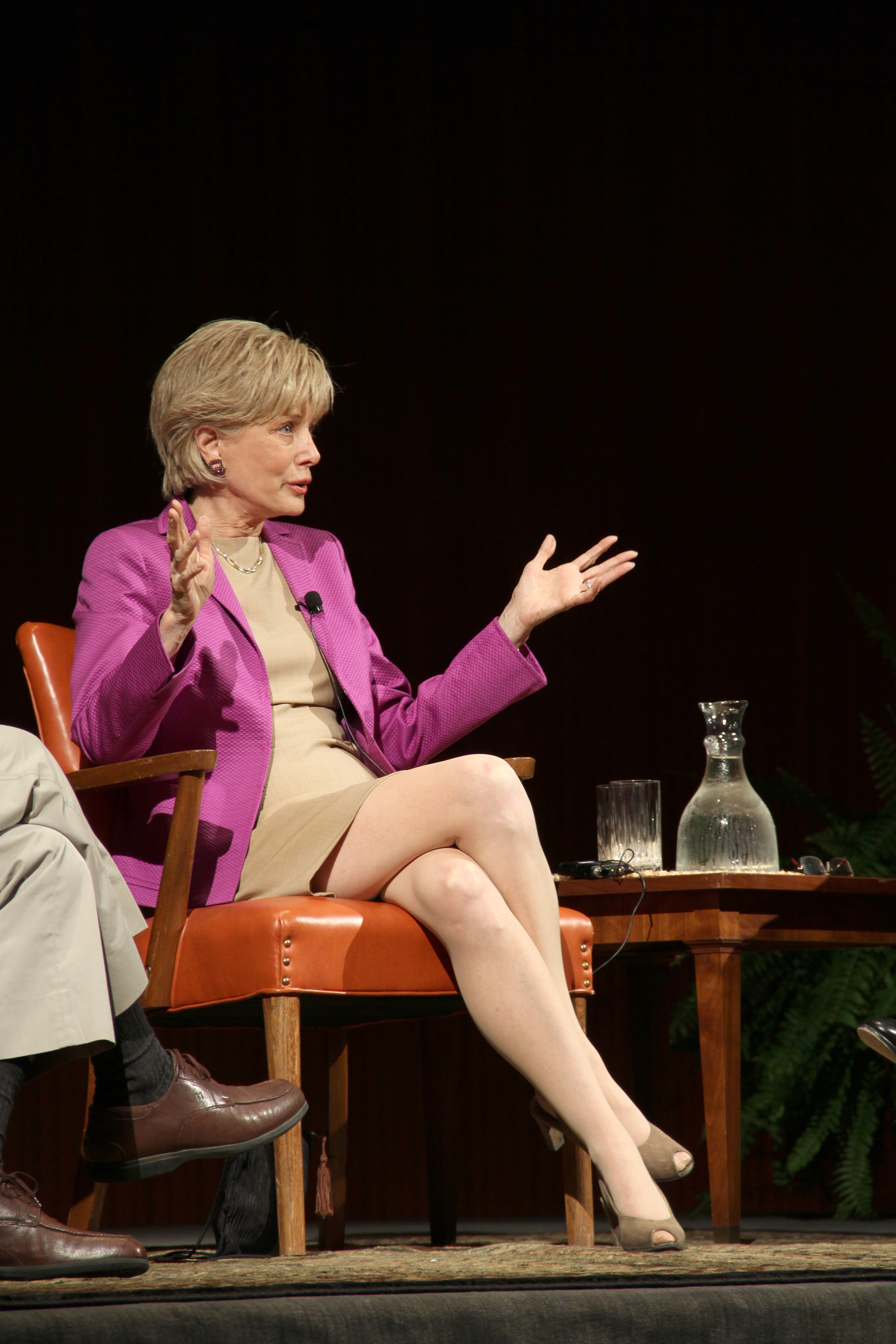An elderly woman, approximately in her 50s or 60s, is seated and appears to be mid-sentence, giving a talk or a speech. She has short blonde hair styled in a "Karen" haircut, and her attire consists of a khaki-colored dress and a pink coat draped over it. A microphone is clipped to her lapel. Her makeup is meticulously done, and she is wearing jewelry. She sits in a brown chair, with her hands raised expressively. To her right, there is a short brown wooden table holding a carafe of water and glasses. On the background, primarily dark, a small plant is visible in the bottom right corner. An additional pair of legs is partially visible on the left-hand side, and just the tip of a shoe can be seen on the right. The overall setting suggests a formal or semi-formal event.